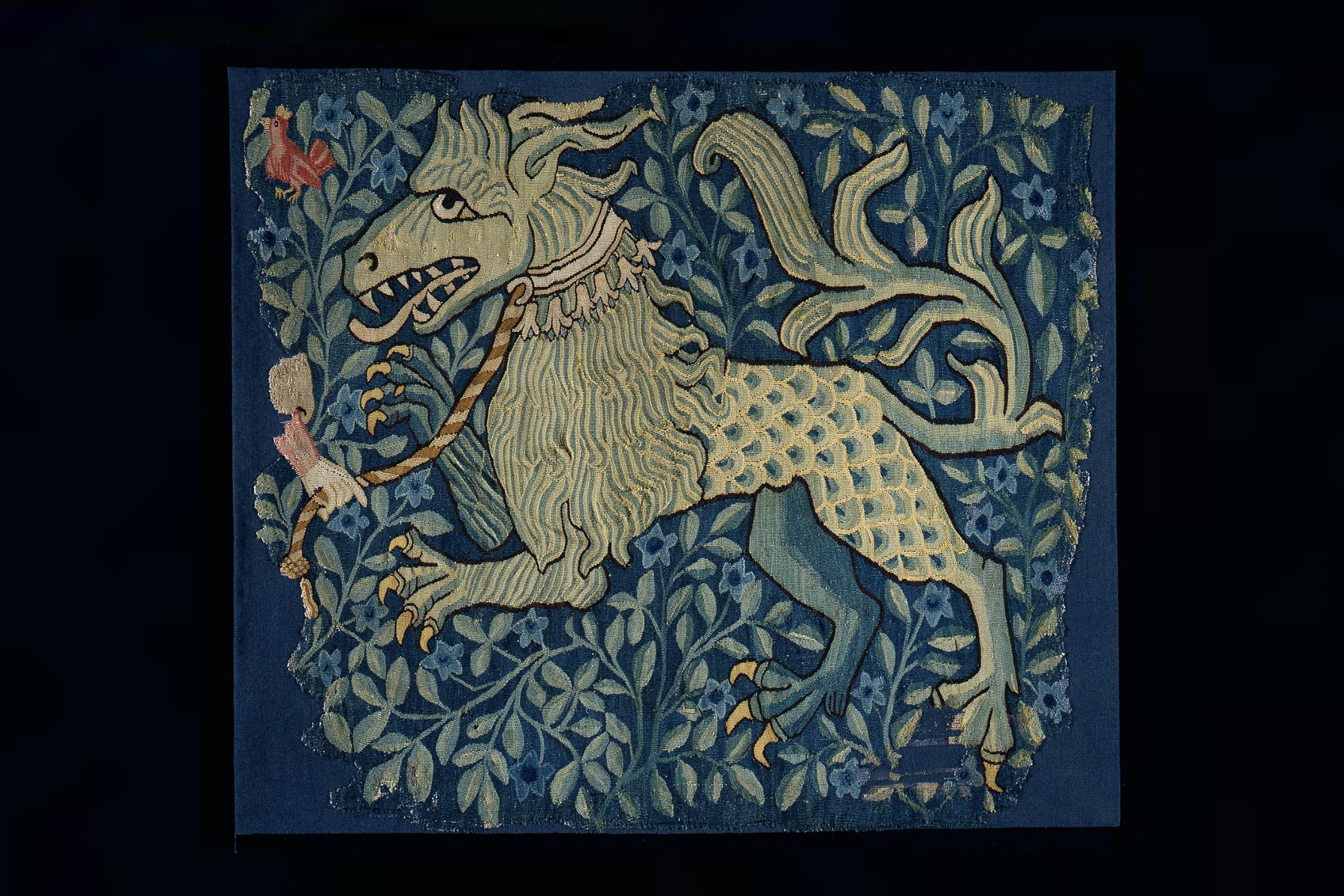The image depicts a detailed, hybrid creature that appears to be a fusion of a lion, dragon, and fish, set against a blue background adorned with numerous flowers and intricate patterns. The creature's head resembles that of a wild and dangerous lion, complete with a mane and sharp teeth, while its body transitions into fish-like scales near the back legs that morph into dragon-like limbs. The creature's lengthy tail, which is unusually long for a lion, ends in tufts of hair and resembles a fishtail. A collar around its neck features hanging, squid-like shapes, and a disembodied hand is holding a leash attached to this collar. The setting includes a red bird with a yellow beak in the top corner, amidst green leaves and blue flowers. This mystical beast is painted with a mix of watercolors, acrylics, or colored pencils on a piece of paper, creating a colorful and surreal composition photographed against a black backdrop.